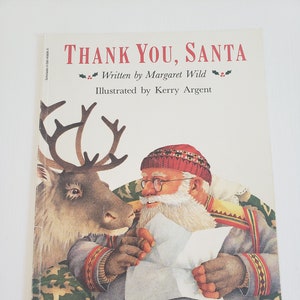The image is a small, square photograph, approximately two inches high by two inches wide, featuring the cover of a Christmas-themed hardback book against a plain light gray background. The book itself occupies most of the image, extending from the bottom nearly to the top. 

At the top of the book cover, "Thank You, Santa" is prominently displayed in bold red letters. Below this title, in black print, are the credits: "written by Margaret Wilde" followed by a small design of three red berries with two holly leaves on either side, and then "illustrated by Kerry Argent," accompanied by a similar holly and berry icon.

The bottom portion of the cover showcases an illustration of Santa Claus seated in a green and gold patterned chair. Santa, who is bearded and wears glasses, is dressed in a yellow, red, and beige sweater with stripes that run across his shoulders and wrists. He holds a piece of paper—likely a list—in his hands. A reindeer with large antlers peeks over the chair from Santa's right side, engaging with Santa as if they are in discussion. Santa also wears a red winter cap and fingerless gloves, adding to the festive detail of the scene.